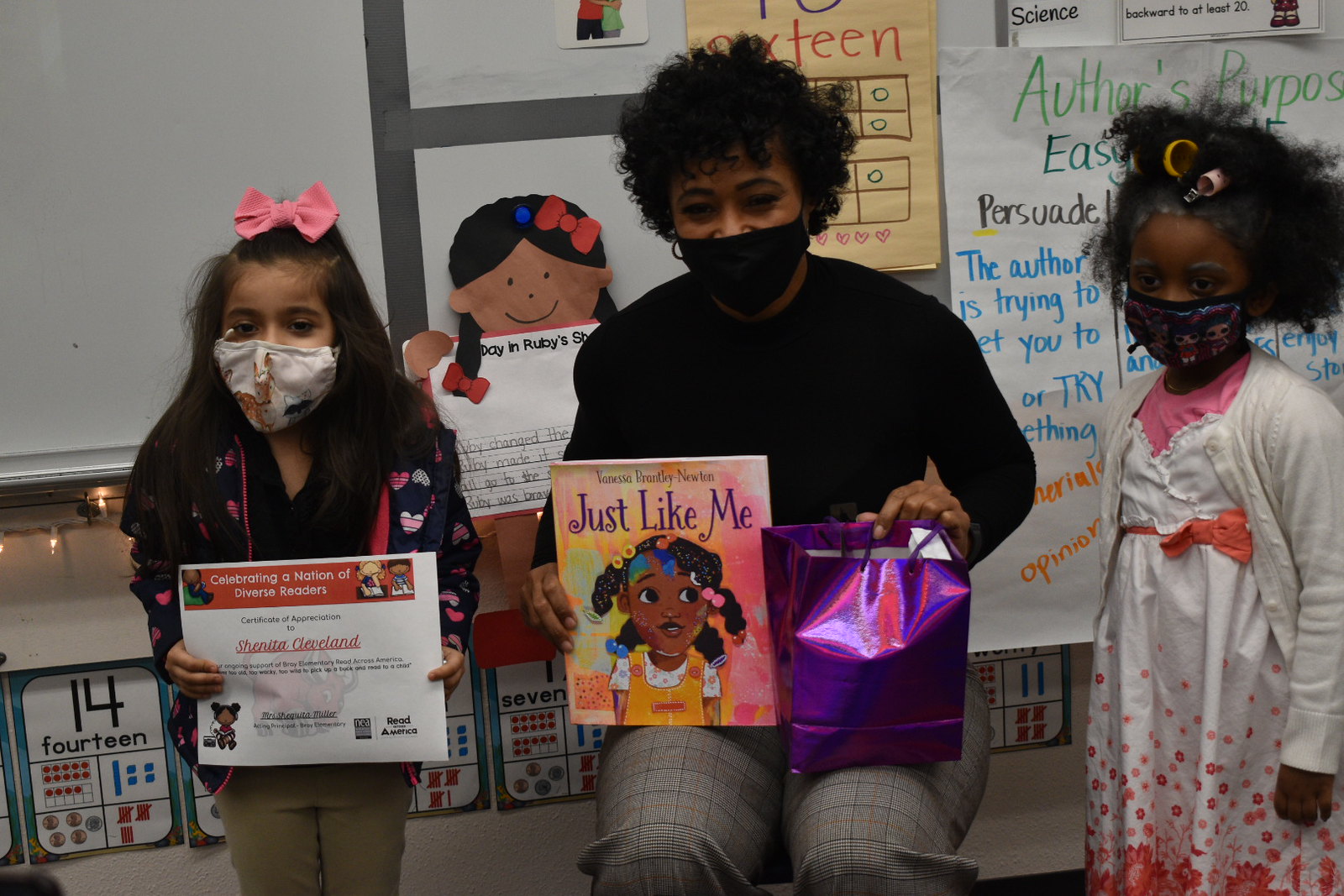This horizontally aligned rectangular photograph captures a moment in a brightly decorated classroom, likely a kindergarten, given the presence of numbers and various drawings and pictures displayed on the walls. At the center of the image is a dark-skinned female teacher, who is seated, wearing gray plaid pants, a solid black long-sleeve top, a black mask, and sporting short curly dark hair. She is holding a brightly colored book titled "Just Like Me," featuring an African-American girl with braids and vibrant hair colors on the cover, authored by Vanessa Bruntley Newton. Additionally, she holds a small, bright purple gift bag.

To the teacher's right stands a young girl with dark skin and messy black hair styled with hair rollers under a dark-patterned mask. She is dressed in a white cardigan over a white dress with coral floral prints and a pink t-shirt underneath. On the teacher's left is another young girl with long brown hair adorned with a pink bowtie, wearing a white patterned mask. She sports a black sweatshirt with pink and white hearts over her outfit and holds a certificate of appreciation that reads, "Celebrating a Nation of Diverse Readers: Shenita Cleveland."

This group appears to be celebrating or recognizing achievements, surrounded by the vibrant and nurturing environment of their classroom.